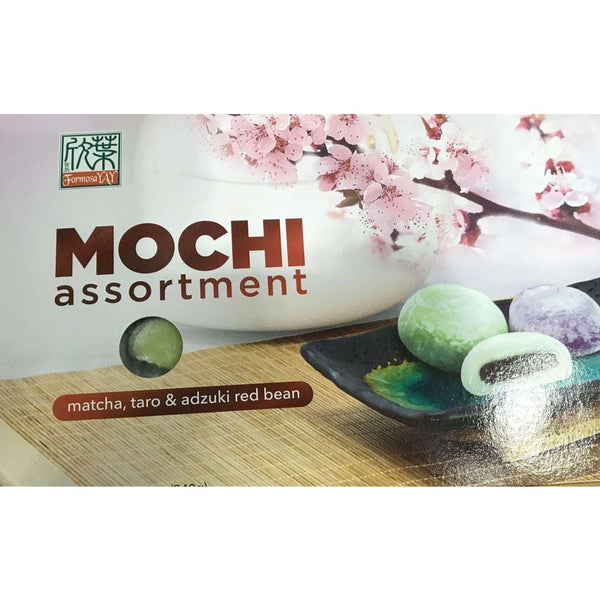The image is a landscape-oriented advertisement for a Mochi assortment, highlighted by a glossy photograph indicative of a light reflection in the bottom right corner. Dominating the view, the product packaging features prominently with the title "Mochi Assortment" written in large, reddish-maroon text. Below this, a green circle and a maroon bar with white text list the flavors: Matcha, Taro, and Adzuki Red Bean. The upper left corner showcases a logo in black, white, and red, presumably reading "Formosa Yay" along with some Japanese characters in green.

The advertisement's bottom half presents a visual setup: a wooden tablecloth surface supports a black plate arranged with the three mochi varieties. One is a perfectly circular lime green mochi, the second is a lavender purple, while the third green mochi is halved to reveal a darker green filling. Above this scene, a cherry blossom branch adorned with pink flowers adds a touch of elegance and cultural context. Overall, the image emphasizes the enticing, hand-held sweet treats positioned against a thoughtfully arranged backdrop, intended to allure potential buyers with its visual and descriptive authenticity.